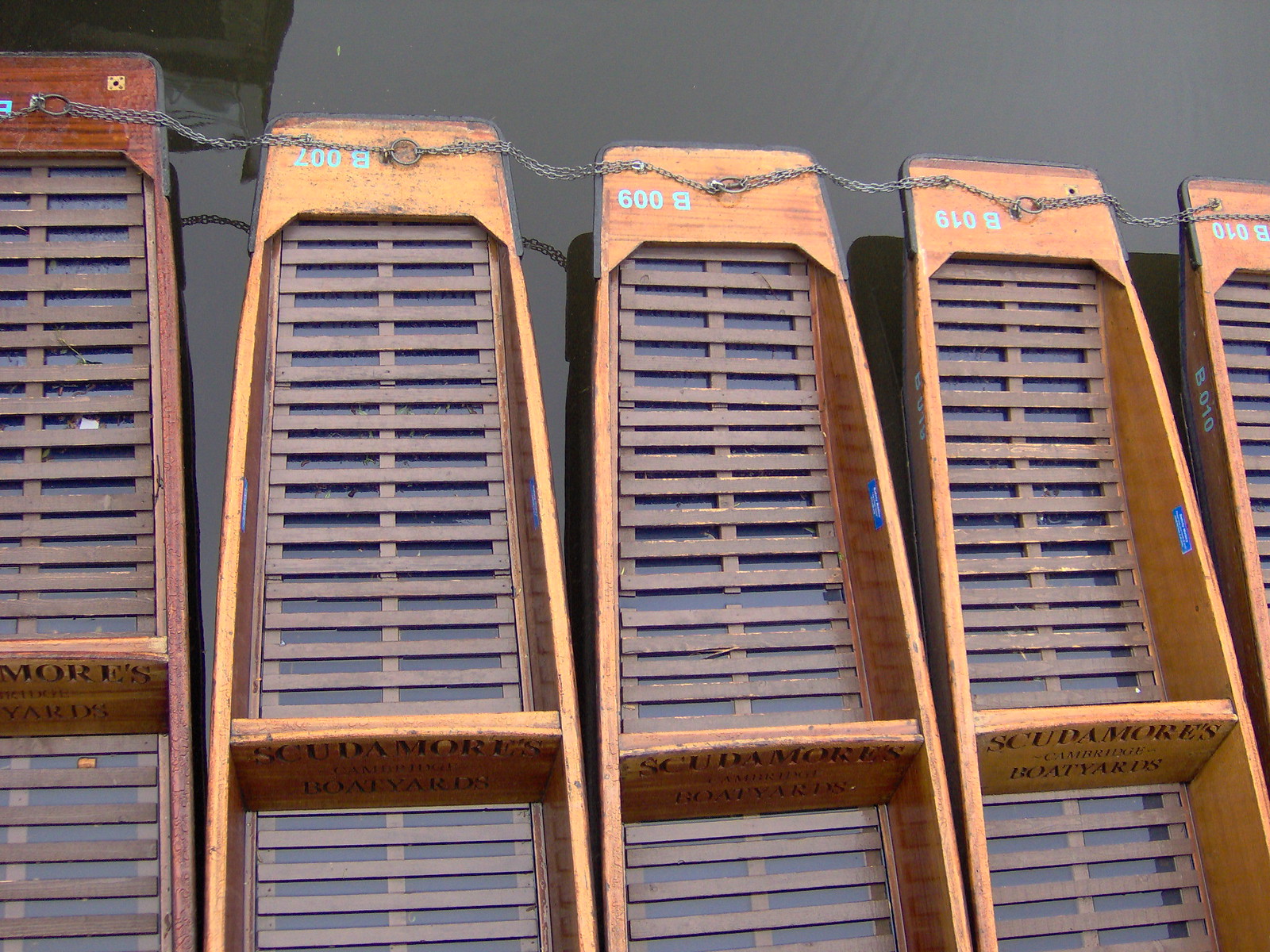The image features five wooden canoes aligned side by side, partially submerged in dark water. Each canoe has a distinctive slatted design at the bottom, giving it an appearance similar to slatted closet doors, yet buoyant. These canoes are connected by a thin chain running along the top. The canoes display identification codes such as B010, B019, B009, and B007, and bear the inscription "Scudamores Cambridge Boatyards" on a wooden plank separating the boat sections. The canoes vary slightly in color, with one being darker brown while the others are lighter wood. A blue sticker or tag can be seen on the front of each canoe. The image appears to be taken from an overhead angle, offering a top-down view of the canoes arranged in parallel.